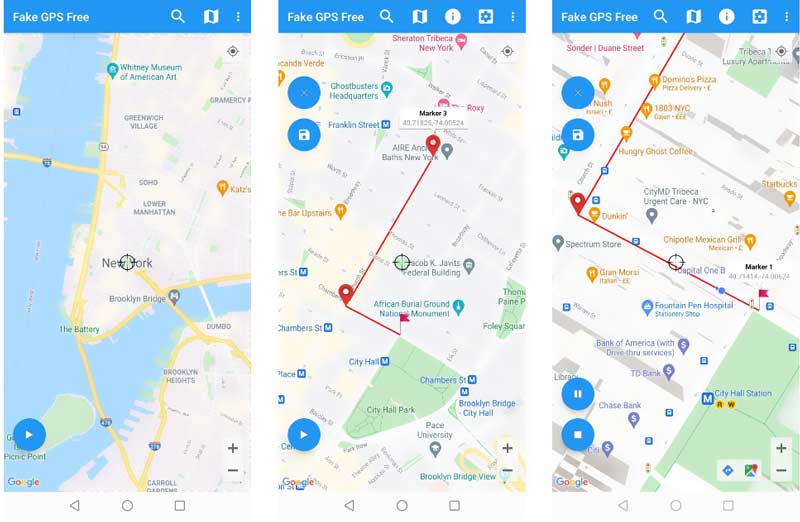The image features three side-by-side screenshots from a GPS application titled "Fake GPS Free," each with a blue header at the top. The app appears to be designed for falsifying location data for potentially deceptive purposes.

1. **Left Screenshot**: The left screenshot displays a map of New York, specifically highlighting the Brooklyn Bridge. The map also shows the surrounding rivers. The blue header contains navigational icons including a magnifying glass, a folded map, and a three-dot menu.

2. **Center Screenshot**: The center image also includes the blue header but with additional icons: an "i" for information and a system preferences icon. The map showcases a more detailed view of an unspecified part of the city with two GPS-mapped lines. One of the lines ends at a flagged waypoint, and other navigational points are also marked, suggesting routes or areas of interest.

3. **Right Screenshot**: The rightmost screenshot provides an even more detailed view of a different location. The header icons are consistent with the previous screens. This view includes more options for map manipulation such as “Close,” “Save to Disk,” and typical media control icons like “Pause” and “Stop,” indicating functionality for recording or managing GPS data.

The app is presented as a tool that could be used for creating mock locations, potentially for dubious purposes such as deceiving others about one's whereabouts. The detailed interface shown in the screenshots provides various controls and settings to manage and save GPS routes.